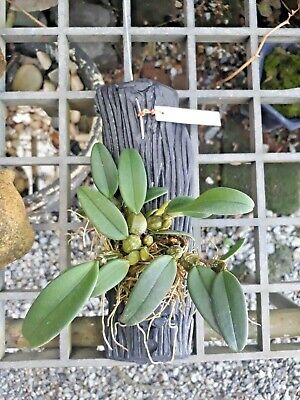In the image, a plant emerges from what appears to be an artificial, gray tree stump designed to mimic wood. The stump serves as a unique holder for the plant, which features numerous green leaves. In the middle of the foliage, there are round, white bulbs that resemble berries, and some strands of moss can be seen around the sides, enhancing the realistic appearance. Attached to the top of the stump is a long white tag. Below, a variety of stones and gravel, in shades of gray, white, and brown, fill a sort of container or pot, adding texture and depth to the scene. In the background, a metal railing with square shapes is visible, with dirt and additional rocks scattered throughout. Small green plants can also be seen in the surroundings, contributing to the natural yet staged composition.